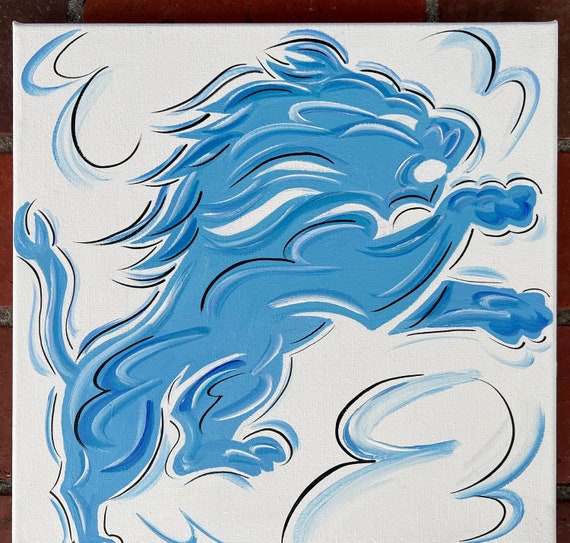This image showcases an artistic rendition of the Detroit Lions logo, presented on a square canvas with a black border. The background is a clean white, adding contrast to the dynamic portrayal of a leaping lion. The lion, primarily depicted in shades of blue with black outlines and white brush strokes, appears to be vigorously jumping, with its head at the top right of the image and its back legs at the bottom left, suggesting a pouncing motion. Energetic swirls and squiggles of blue and black around the lion accentuate the sense of vigorous movement, while the lion’s mane is rendered with expressive blue and white streaks. The image has a cloudy, almost ethereal quality, evoking the floating imagery of a Greek god’s cloud, enveloping the lion in a mystical aura. The artistic execution suggests a hand-painted or hand-drawn technique, emphasizing the fluid and dynamic nature of the iconic emblem, with no text or additional details in the background.